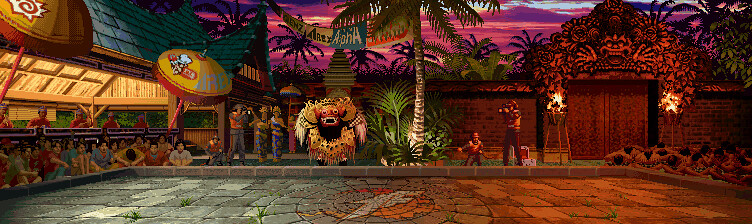A vibrant screen capture from a video game or computer game, showcasing a vividly detailed Polynesian setting. The scene centers around a fighting pit, bordered by contrasting hues: the right side bathed in browns, and the left side dominated by grays and blues. On the right-hand side, groups of men are seen bowing down. A prominent stylized 'F' is positioned at the lower center of the image, potentially indicating a significant game element.

To the left, an ornate gate with a stylized arch looms, embellished with vibrant flames. A stately palm tree stands at the center, its silhouette connecting to the roof of a Polynesian-style building with a striking blue roof adorned with unreadable lettering. Adjacent to the palm tree, a large creature with a brown and tan color scheme gazes ahead.

The scene is bustling with spectators; numerous figures are shown seated in front of the blue-roofed building, keenly watching the unfolding events in the fighting pit. A large, yellow umbrella with inscribed letters provides some shade. In the backdrop, a mystical purple sunset adds to the atmospheric setting, casting a serene glow over the arch and gate. The entire image is framed within a rectangular border, capturing the vibrant, immersive world of the game.